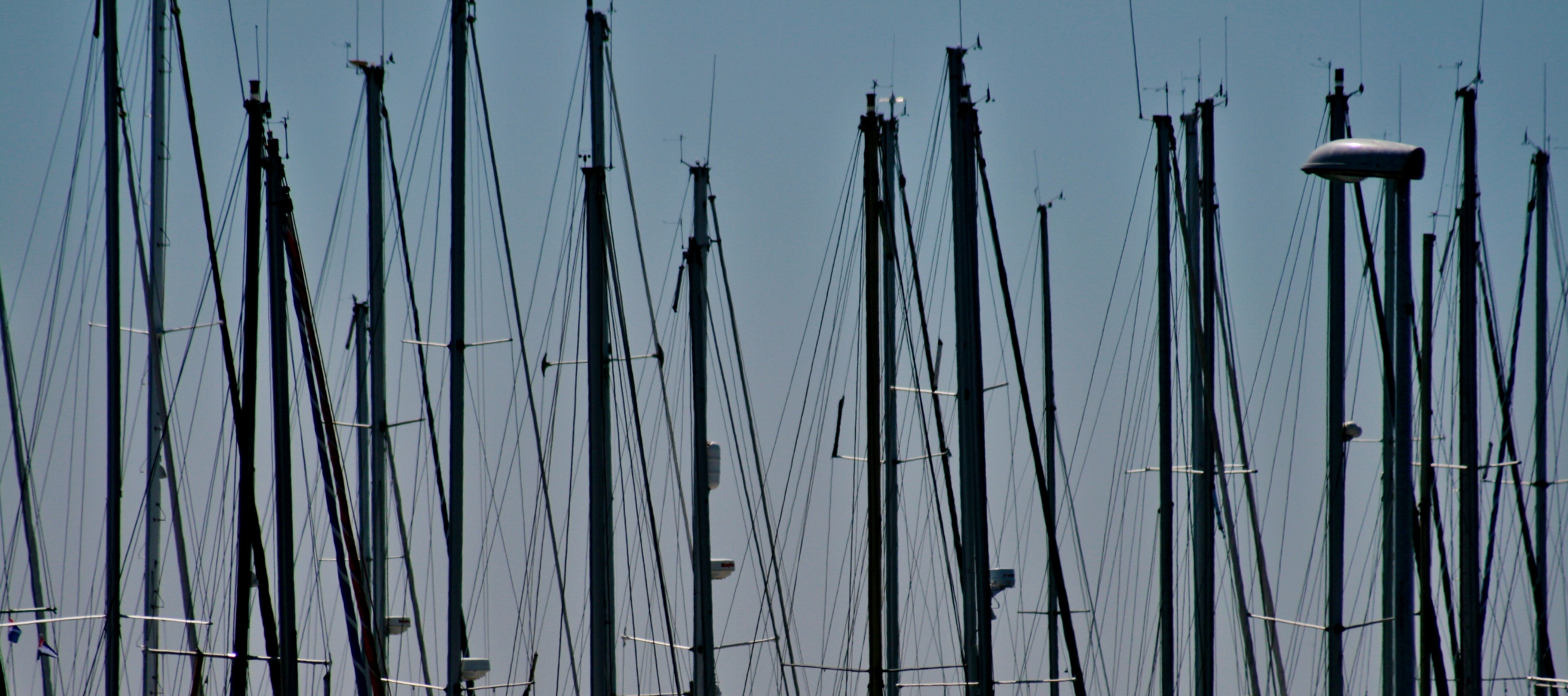The photograph captures a clear, cloudless blue sky above a forest of sailboat masts, densely packed together, likely at a shipyard or harbor. The masts, which are dark black or deep blue, are prominently vertical poles with thin, guide wires extending from their tops and sides. There are no sails attached to any of the masts, leaving only their skeletal structures visible. The masts vary in height, with some being exceptionally tall and others shorter, but most of them extend about three-quarters of the way up. The scene is dominated by these linear, A-frame-like structures, densely clustered, giving the impression of well over twenty sailboats lined up next to each other. In the foreground, one of the masts features an unusual long black object at its tip, adding a unique detail to the otherwise repetitive pattern of poles and wires set against the expansive, azure backdrop.